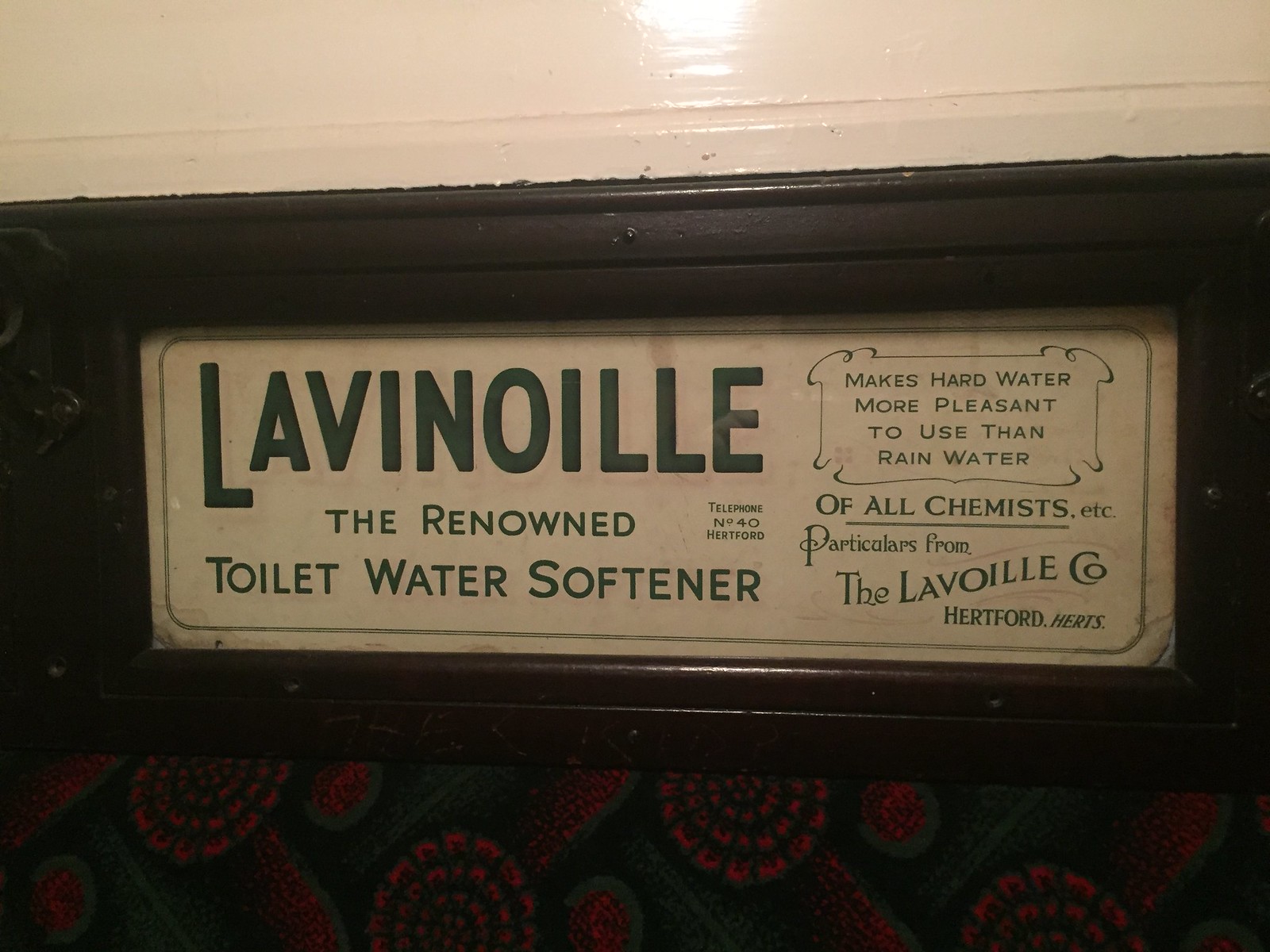This image depicts an old, rectangular sign encased in a dark wood frame, likely dating back to the 1930s or 1940s. The sign, which has an off-white, beige-colored background, features forest green lettering with a heading that reads "LavinOil, The Renowned Toilet Water Softener." To the right side of the sign, there's a smaller square with a decorative border containing the phrase, "Makes hard water more pleasant to use than rainwater". Below this square, it states, "Of all chemists, etc. Particulars from the Lavioil Company, Hartford Hertz," and lists a contact detail as "Telephone Number 40 Hartford." The sign is mounted on a white wall, and below it, a brown wooden ledge is visible. Despite its age, noticeable from the weathered and scratched frame, the sign retains its vintage charm.